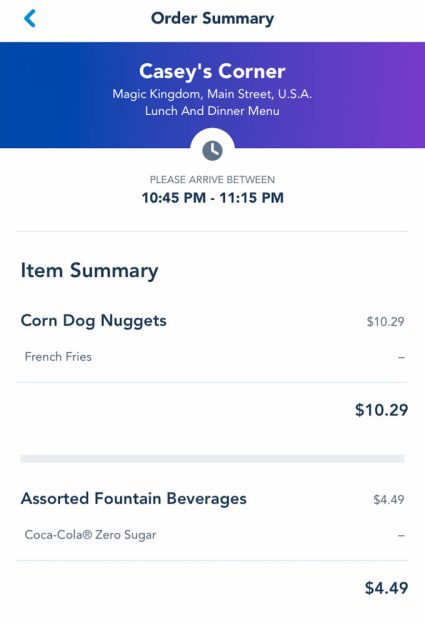This is a screenshot from an unidentified app featuring an order summary. At the top left, a blue arrow points to the left next to the header "Order Summary." A banner, which transitions from dark blue on the left to light purple on the right, prominently displays in white text: "Casey's Corner, Magic Kingdom, Main Street USA, Lunch and Dinner Menu." Below this banner, a clock face icon is present with the text: "Please arrive between 10:45 PM to 11:15 PM."

The "Item Summary" section follows, listing "Corndog Nuggets, French Fries" priced at $10.29, with the total for this item repeated as $10.29. The list continues with "Assorted Fountain Beverages," priced at $4.49, specifically noting a "Coca-Cola Zero Sugar." The price for the beverages is repeated below as $4.49. 

The screenshot is devoid of any photographic elements, people, animals, plants, flowers, trees, buildings, automobiles, motorcycles, bicycles, or airplanes. The image is purely text-based, centered around the detailed menu and order specifics.